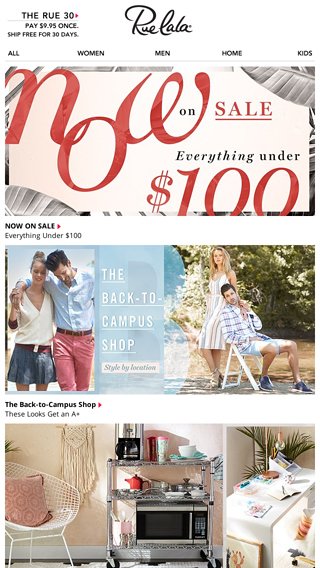This image is a screenshot from a shopping website, featuring various promotional segments and navigation options against a white background. At the top, black text reads "THE RUE," adjacent to a red arrow pointing to the right. Below, it states, "Pay $9.95 once, ship free for 30 days." Centrally displayed is the phrase "Ooh, la la."

Continuing downward, the categories "All," "Women," "Men," "Home," and "Kids" are listed. A prominent graphic declares, "Now on Sale: Everything Under $100," accompanied by a red arrow and set against black text.

The next graphic showcases a couple walking and another scene with a man seated in a chair with a woman standing behind him. It is labeled "The Back to Campus Shop, Styled by Location," on a pale blue background with white text, complemented by the tagline, "These looks get an A+," in black text with a red arrow pointing right.

Further down, another graphic appears, depicting a kitchen setting. It includes a beige wall, a cart holding a microwave and a coffee pot, and a white wire chair with a cushion.